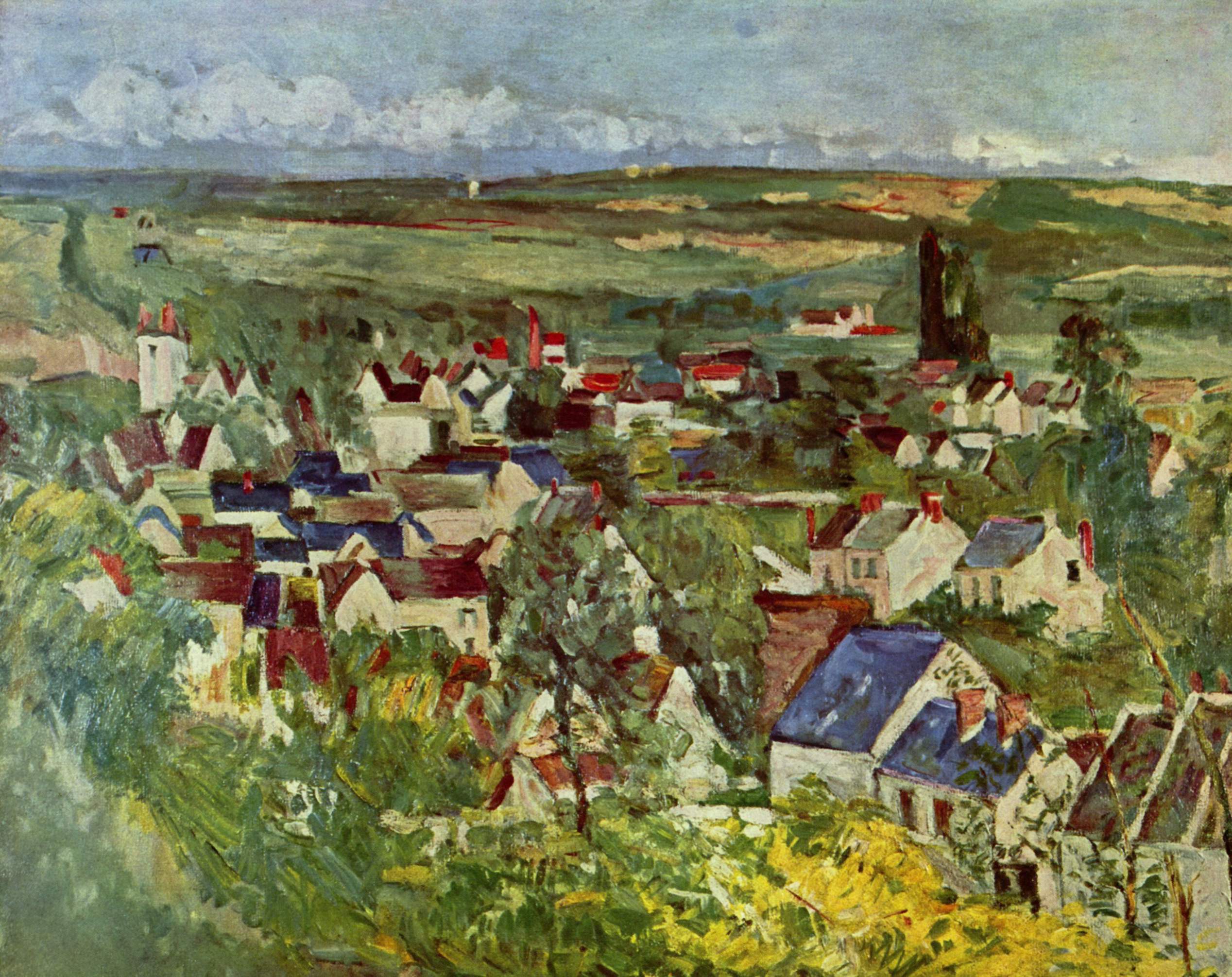The image depicts an oil-based painting of a rural village set within a picturesque countryside. The scene features 20-25 small cottages nestled in a valley surrounded by rolling green hills and a cloudy blue sky. The houses are characterized by their colorful rooftops, with an array of blue, red, and tan shades. Notably, there is a house in the lower right corner with two distinct peach-colored chimneys, while six or seven other houses sport red chimneys. The village exhibits a serene landscape void of people, animals, or vehicles, emphasizing its tranquil, almost timeless nature. The foreground is dominated by the quaint cottages and their chimneys, while the background transitions into expansive farmland with scattered trees, shrubs displaying splashes of purple and yellow, and subtle traces of footpaths rather than developed roads. The detailed rendering of the hills and clouds alongside the simpler depiction of the village creates a harmonious balance, capturing the essence of rural life, reminiscent of a Norman Rockwell scene.